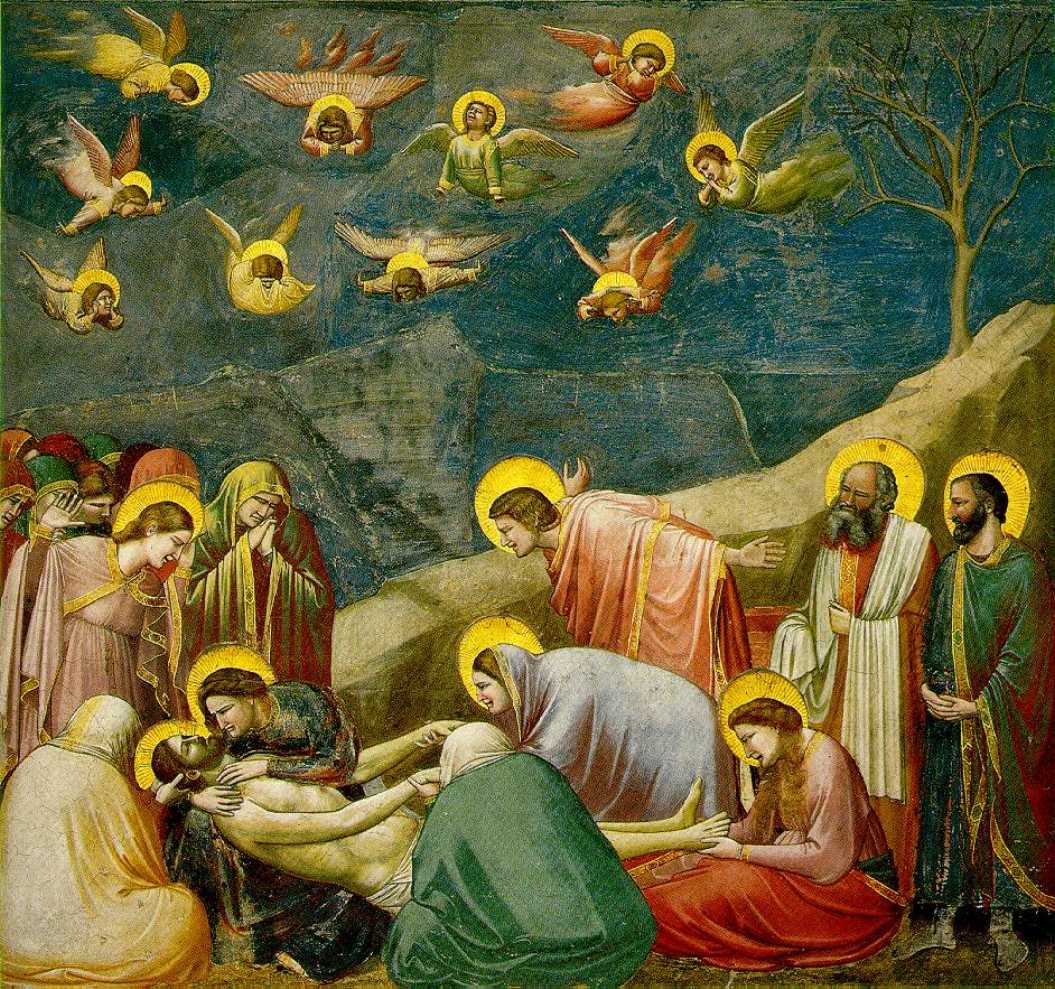This detailed drawing, possibly from the 17th century or earlier, depicts a poignant religious scene centered around Jesus, who lies lifeless on the ground, leaning against a support. Surrounding him are numerous figures, all with golden halos indicating their holy status, including wise men, women, and angels. The women closest to Jesus are dressed in long gowns of varying colors. One woman in a red dress is at his feet, holding them tenderly. Another woman with a white gown and shawl bends over Jesus, while a third woman leans in close. Among them, some women appear to be mourning, standing or kneeling, adorned with these golden halos. In the sky above, a dark turquoise background highlights the presence of about ten small angels, painted with wings and golden halos, creating a sense of divine observation. To the right of the scene, a leafless tree stands against a brick wall, while in the background, three wise men with beards and long gowns watch over the solemn gathering. The image is filled with vibrant colors such as greens, reds, yellows, and golds, enhancing the emotional and spiritual depth of the depiction.